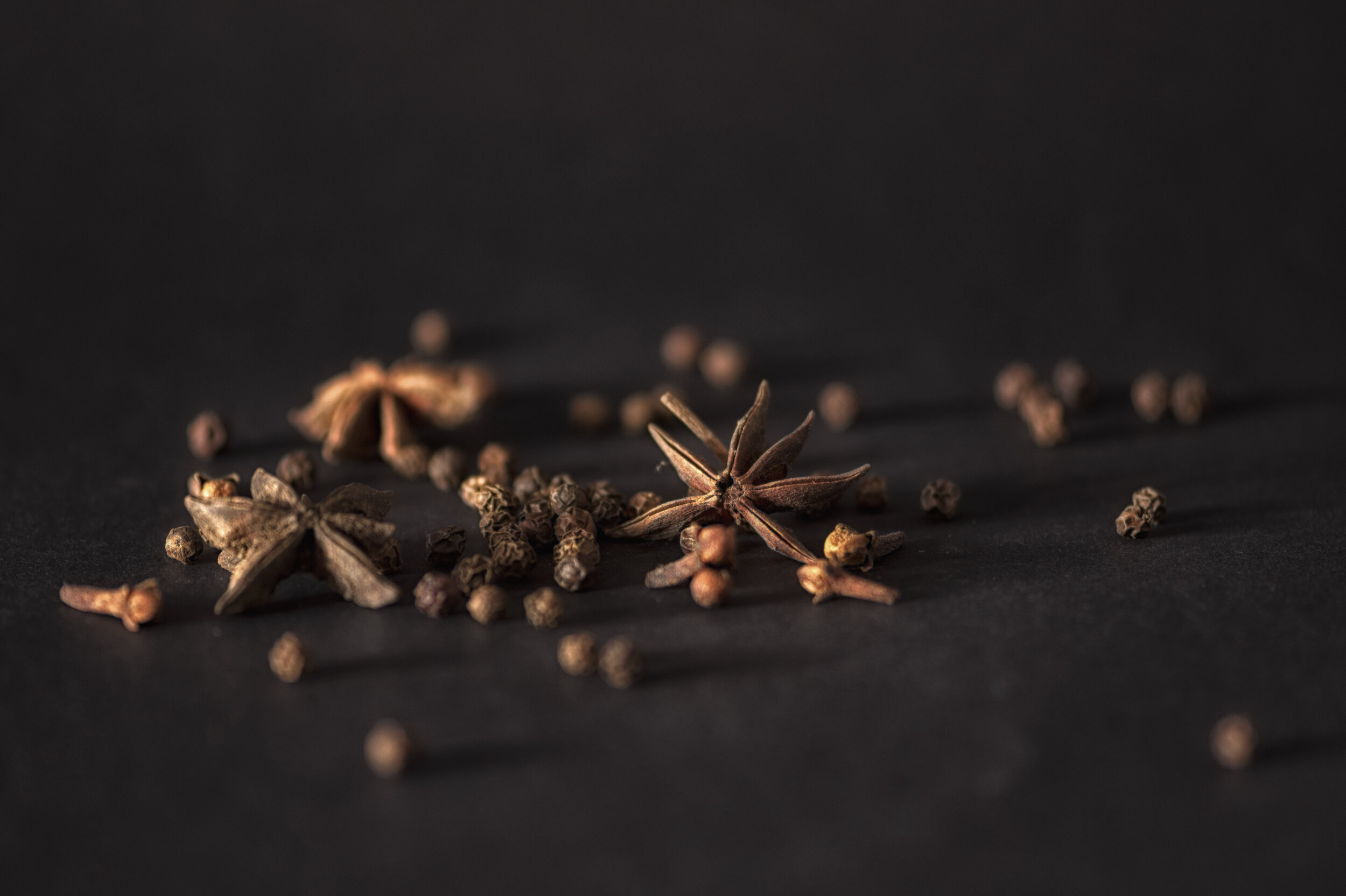The image features a predominantly black background, transitioning to lighter gray tones. The main focus is a narrow band in the center, showcasing what appears to be dried star anise. Two prominent star anise pods dominate the foreground, with one slightly out of focus in the background. Scattered around are smaller, round seed-like structures, roughly pea-sized, which further enhance the plant-like nature of the composition. The star anise pods exhibit a starfish-like shape with several petal-like spokes and a brown to goldish-orange hue. The background elements remain blurred while the central seeds and pod details are in sharp focus, creating a vivid contrast against the dark backdrop.